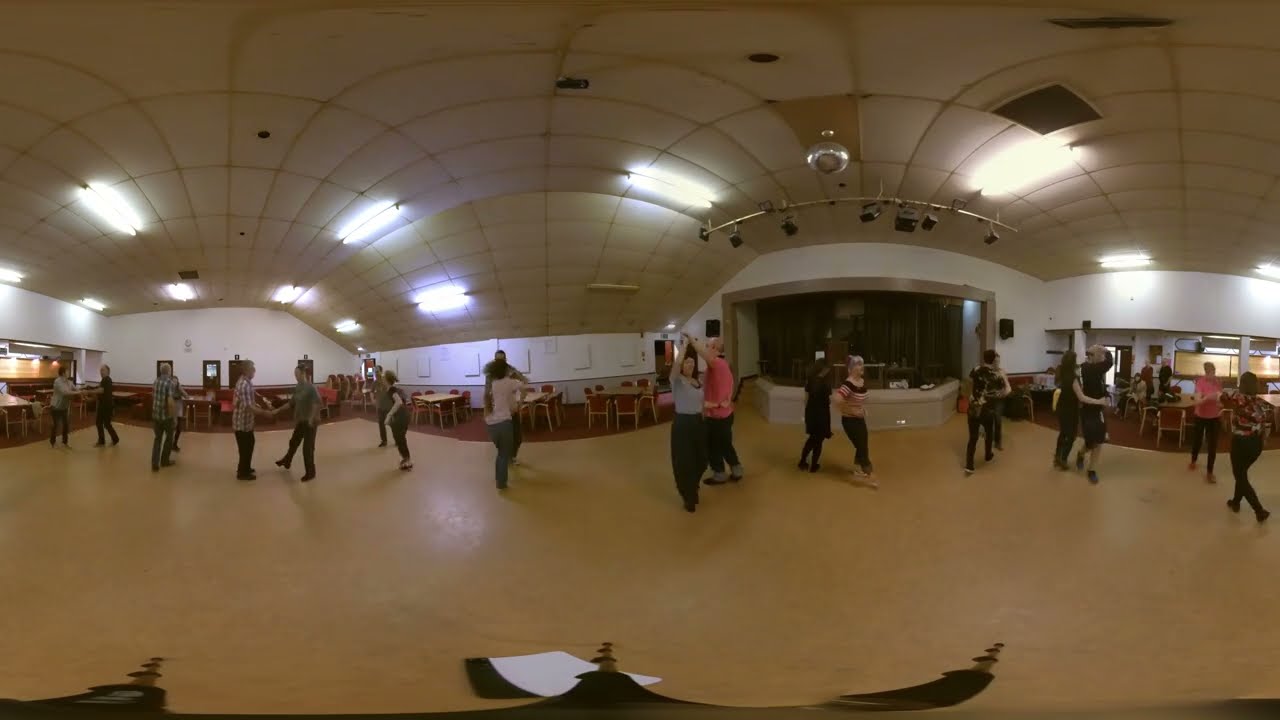The image appears to be a panoramic or 360-degree photograph of an indoor dance hall, possibly a community center. The image is somewhat distorted, giving a rounded and warped appearance, likely due to the type of camera used. The main focus is a large, smooth, light brown dance floor, which occupies the center of the image. Around the dance floor, there is burgundy carpeting with brown tables and red chairs arranged around it.

In the photograph, numerous couples are engaged in what seems to be a ballroom dancing class. Each couple is at different stages of their dance, with some twirling and others holding hands in dance positions. The dancers, who appear to be of Caucasian descent, are dressed in casual attire.

A white-tiled ceiling with fluorescent lights and a disco ball hangs above the dance floor. To the right of center in the image, there is a white stage with the lights turned off. The walls of the hall are white, further enhancing the bright and open atmosphere of the space.